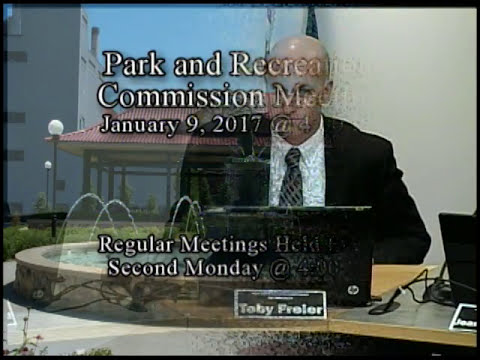The image appears to be a low-resolution screenshot from a video, capturing the transition between two scenes. The first scene is an establishing shot of an administrative building, featuring a round concrete fountain in the courtyard. Overlaid text, partially obscured due to the transition, reads "Parks and Recreation Commission Meeting January 9th, 2017" followed by "Regular meetings held second Monday at 4 p.m." The transition fades to a scene featuring a bald-headed man identified by a nameplate as Toby Freeler or Toby Preeler, seated behind a desk with an HP laptop open in front of him. Toby is wearing a black suit, a white button-up shirt, and a striped tie in shades of black and gray. Due to the merging text, his face is somewhat obscured. The overall scene suggests Toby is participating in the mentioned Parks and Recreation Commission meeting. There is also a reflection on the glass showing the fountain outside, further linking the two scenes.